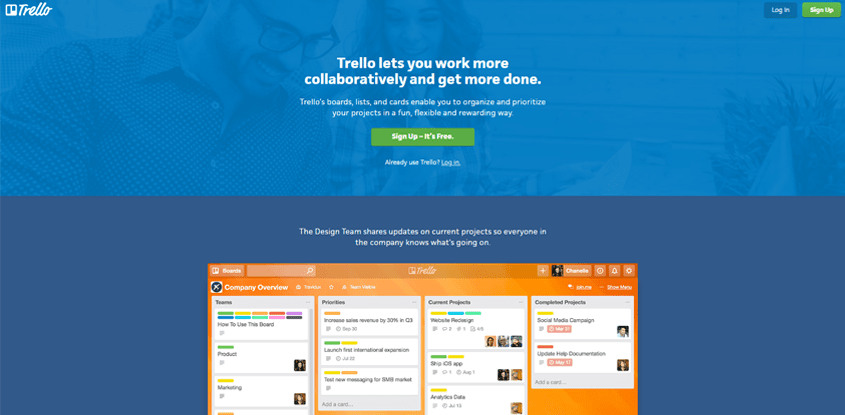This is a screenshot of the Trello homepage. The page is distinctly divided into two background colors: the top half features a bright blue backdrop, while the bottom half has a navy blue background. In the upper left corner sits the Trello logo and the word "Trello" in a casual white font. The logo resembles a square box with one of its quadrants in white.

On the far right side of the top section are two buttons: a navy blue "Log In" button and a green "Sign Up" button. Centered at the top of the page is the headline "Trello lets you work more collaboratively and get more done" in bold white text. Directly below this, a fainter white text reads, "Trello's boards, lists, and cards enable you to organize and prioritize your projects in a fun, flexible, and rewarding way."

Further down is a prominent green "Sign Up – It's Free" button, followed by a prompt in white text that says "Already use Trello? Log in." 

Transitioning to the bottom half of the page with a navy blue background, there is a piece of faint, tiny white text at the top that states, "The design team shares updates on current projects so everyone in the company knows what's going on." Below this is a small horizontal orange box with a search bar at the top. The box features the Trello name in the middle alongside notification icons and a user profile picture and name. To the left of this box in white text, it reads "Company Overview."

The navy blue section is partitioned into several vertical columns of information, each housed within its own rectangular box.